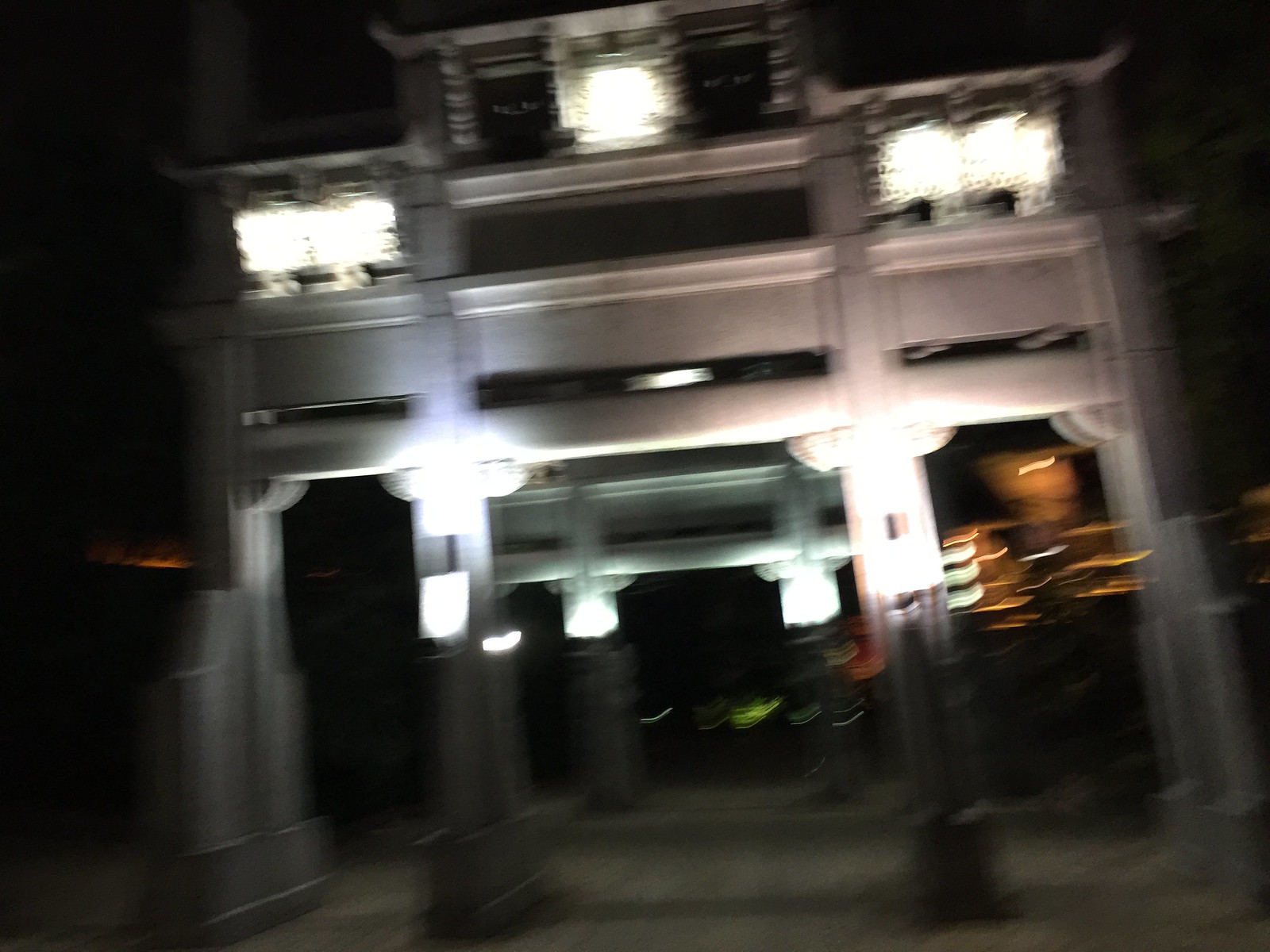This photograph depicts a large, tan and white, metal structure that appears to be an entrance gate, possibly leading into a Chinatown or similar area. The image is taken at night and is highly blurry with a noticeable shaken effect, indicating the camera was moved during the capture. The structure is illuminated with multiple white lights at the top and bottom, which appear distorted and give off a warped "warp drive" look due to the blurriness. 

The gate itself seems to incorporate a rectangular shape with prominent metal bars and columns, forming three doorways, with the central doorway being the widest. The ground in the photo is concrete and slopes from the bottom right corner to the left. In the backdrop, additional lights from other buildings are seen. These lights vary in color from subtle red and green to more intense yellow or orange, all appearing as squiggly lines due to the motion blur. The photograph is set against a black sky, accentuating the illuminated elements of the structure and surroundings while keeping other details obscured in the darkness.